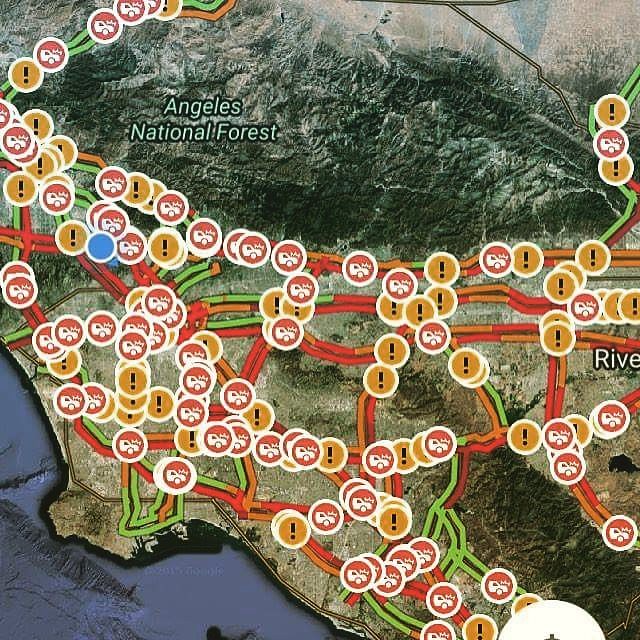This image is a detailed color map, likely a screenshot from Google Maps, depicting the southern California region, specifically highlighting the Angeles National Forest prominently in the upper right corner. The map shows various roadways with the primary focus on traffic conditions. Roads across the map are colored green, orange, red, and light orange to indicate different levels of traffic flow, with green representing smooth traffic and red indicating significant congestion. Scattered across the map are numerous symbols: red circles with a white border and a car graphic signifying car accidents, and yellow circles with a black exclamation mark indicating incidents or warnings. The map also features a white circle with a blue dot, probably indicating the viewer's current location. The satellite view reflects diverse terrain, including lush green mountains near the top right, transitioning to tan desert areas, with the lower left section showing a blue expanse suggestive of a large body of water or ocean. The complex layout and numerous symbols underscore heavy traffic and frequent accidents in the region.